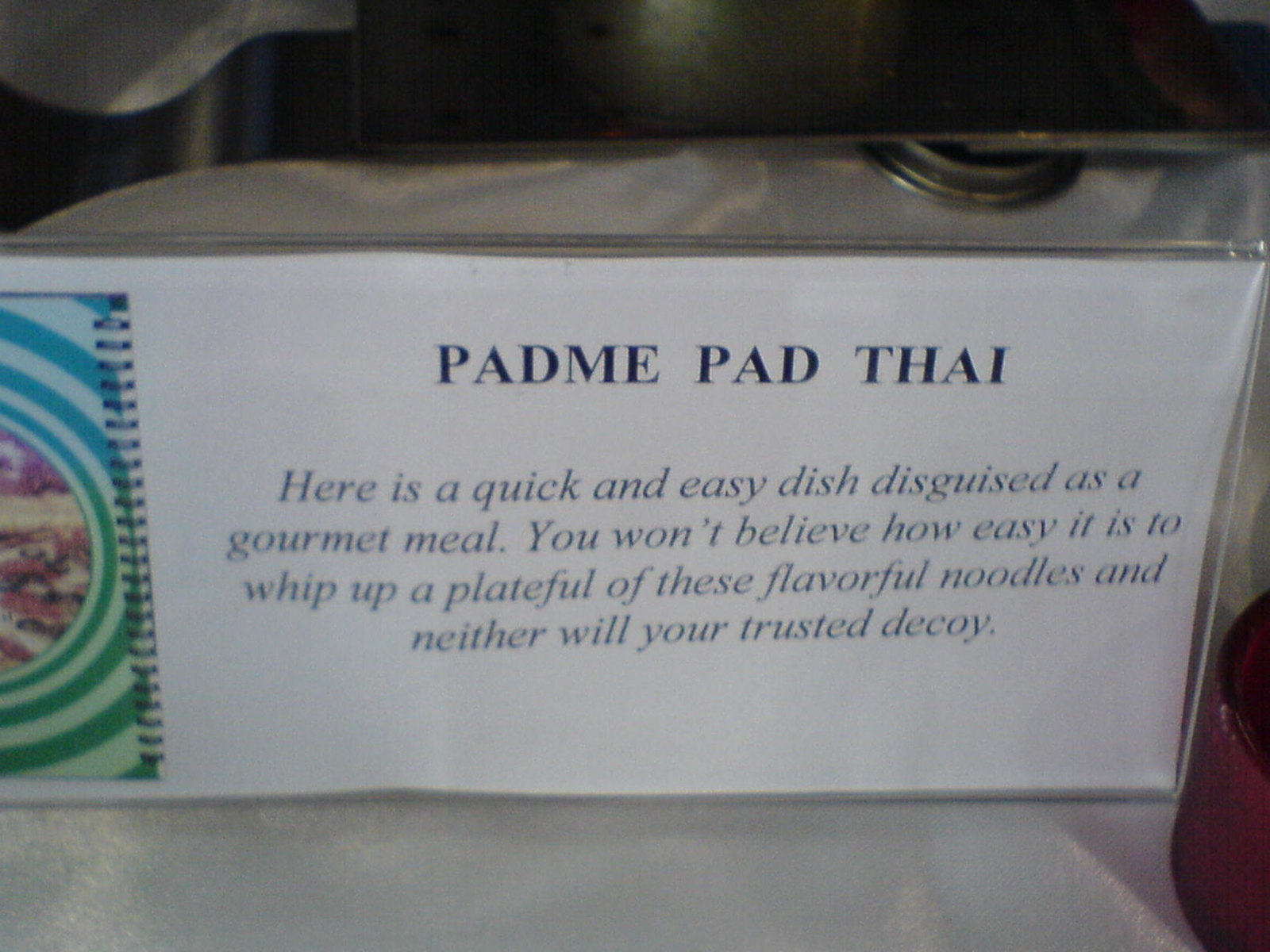The image depicts a page from a recipe book set on a white tabletop. The page prominently features black text that reads, "Pad Mee Pad Thai" in all capital letters. Below the title, a description reads, "Here is a quick and easy dish disguised as a gourmet meal. You won't even believe how easy it is to whip up a plateful of these flavorful noodles, and neither will your trusted decoy." To the left of the text, there is a partially visible binder and a picture of the Pad Mee Pad Thai dish, adorned with a border of light and dark blue circles fading into light and dark green circles. The page appears to be laminated with a small clear border. In the background, there’s a hint of a white tablecloth, a red object to the right, possibly a register screen, and a candle, adding to the overall setup.